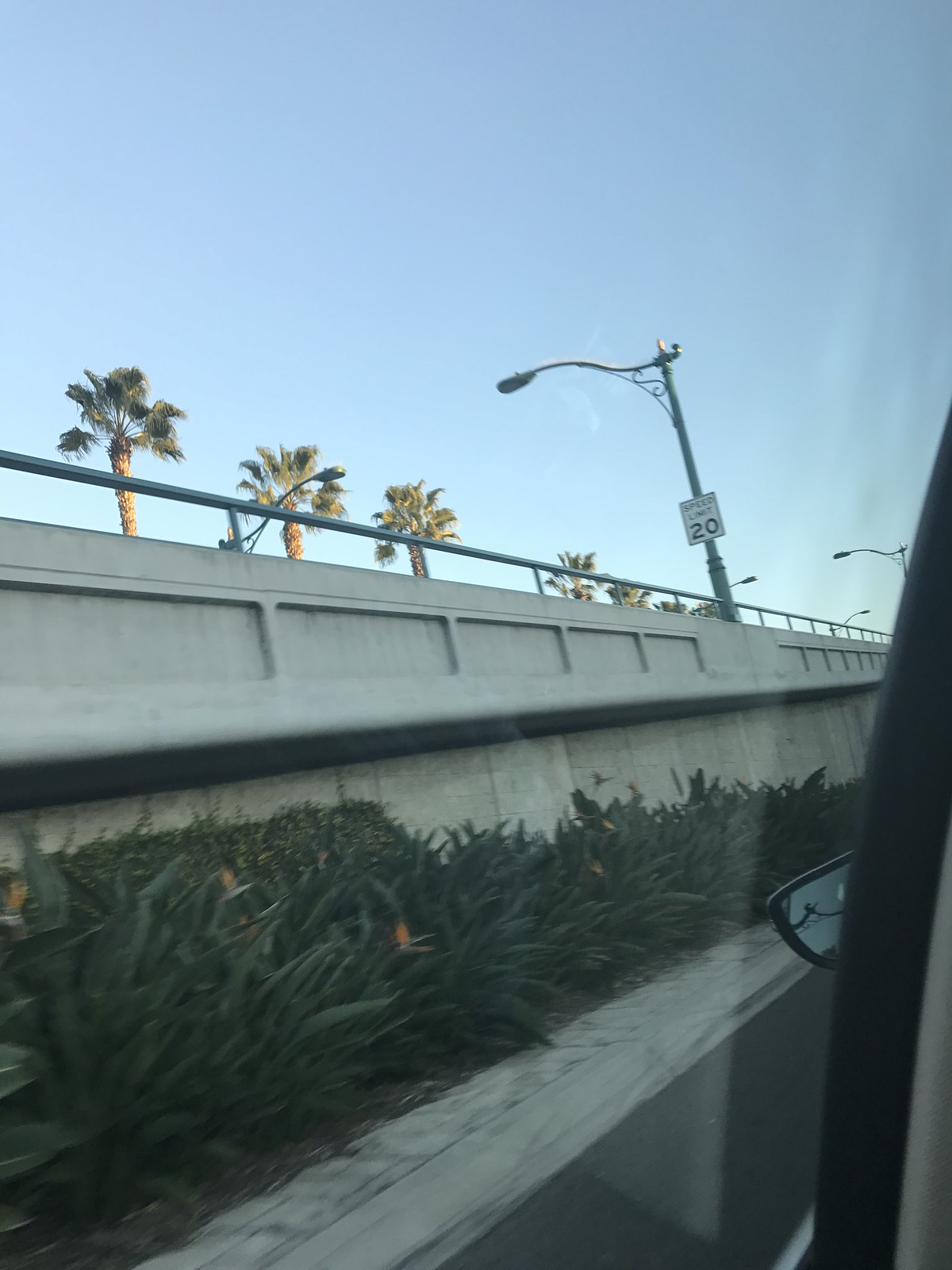This outdoor photograph, captured from the passenger side of a vehicle, looks out of the window and slightly upward to the left. The perspective is angled over a concrete wall barrier, revealing a speed limit sign atop a lamppost. This sign, positioned above the barrier, indicates a speed limit of 20 mph, suggesting the presence of another road beyond the visible wall. In the distance, five elegant palm trees with lush green fronds rise against a backdrop of clear blue skies, evoking a serene, sunny day.